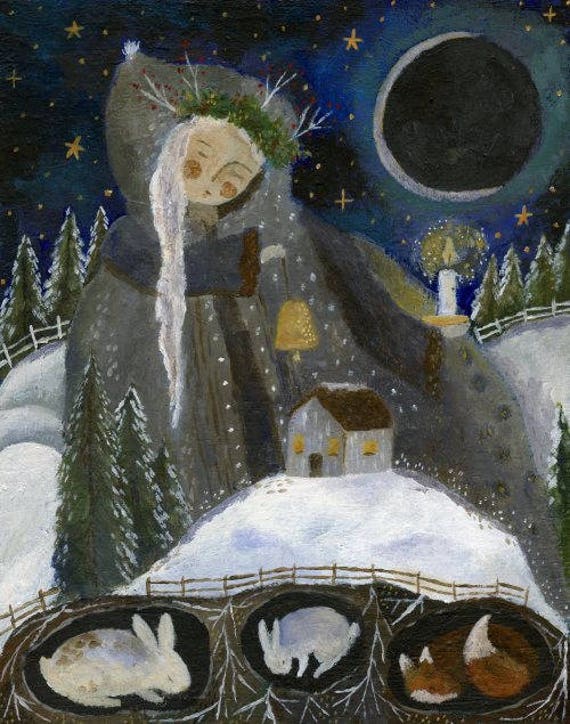This exquisite oil painting, likely digital in nature, portrays an impressionistic Christmas scene rendered in portrait mode. Dominating the composition is a towering woman, possibly an embodiment of Mother Nature, adorned in a gray fur coat interwoven with images of frosted pine trees. Her voluminous white hair cascades down as she holds a golden bell aloft with her left hand and a lit white candle with her right over a small, brown-roofed barn nestled on a snowy mound. The barn features three glowing yellow windows, amplifying the warm, festive ambiance.

Beneath the snow-capped mound, a cozy subterranean world reveals itself, showing hibernating animals in their nests: three bunnies—a white rabbit with brown spots, another purely white, and an orange fox with a contrasting white tail and ears. The scene is encircled by a simple wooden fence.

The backdrop is a mesmerizing dark blue starry sky, punctuated by glimmering golden stars and anchored by a moon with a delicate crescent. In the distance, more pine trees stand tall, encapsulating the serene essence of a winter night, making this image reminiscent of a heartfelt Christmas card.